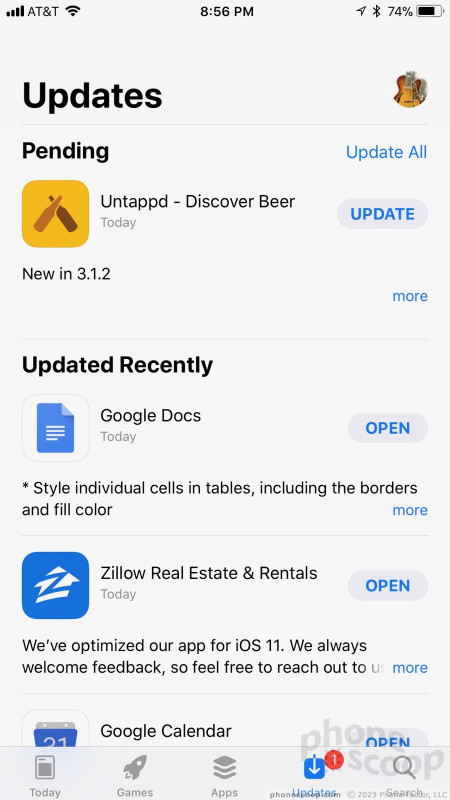Screenshot of a smartphone update screen, displaying pending and recently updated applications. At the top of the screen, the status bar shows signal strength icons for AT&T, a Wi-Fi indicator, the time (8:56 p.m.), a directional triangle Bluetooth icon, and the battery level at 74%. Below, in bold black text, the section titled "Updates" is displayed on the left, accompanied by a circular profile image featuring a guitar on the right.

The section for pending updates shows an app titled "Untappd - Discover Beer," identified by a yellow square icon with two crossed beer bottles. An oval "Update" button is positioned to the right of this app listing. Additionally, there is a section labeled "Updated Recently" listing two newly updated apps: "Google Docs" and "Zillow Real Estate & Rentals."